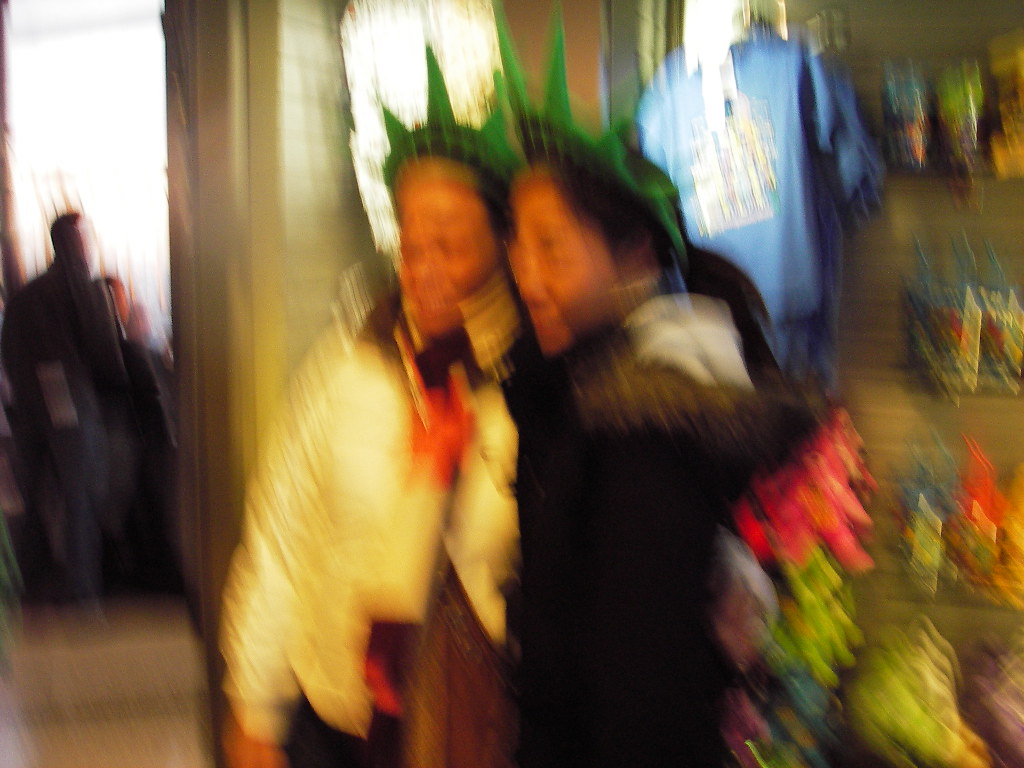In a slightly blurred photograph taken inside a quaint gift shop, two individuals stand closely together as if posing for a picture. They are facing towards the lower left of the image, which cuts off some of their front details. Both individuals are adorned with green headbands resembling the crown of the Statue of Liberty. The person on the left is dressed in a white coat, while the person on the right sports a black one. Various trinkets and souvenirs typical of a gift shop can be seen in the soft-focus background.